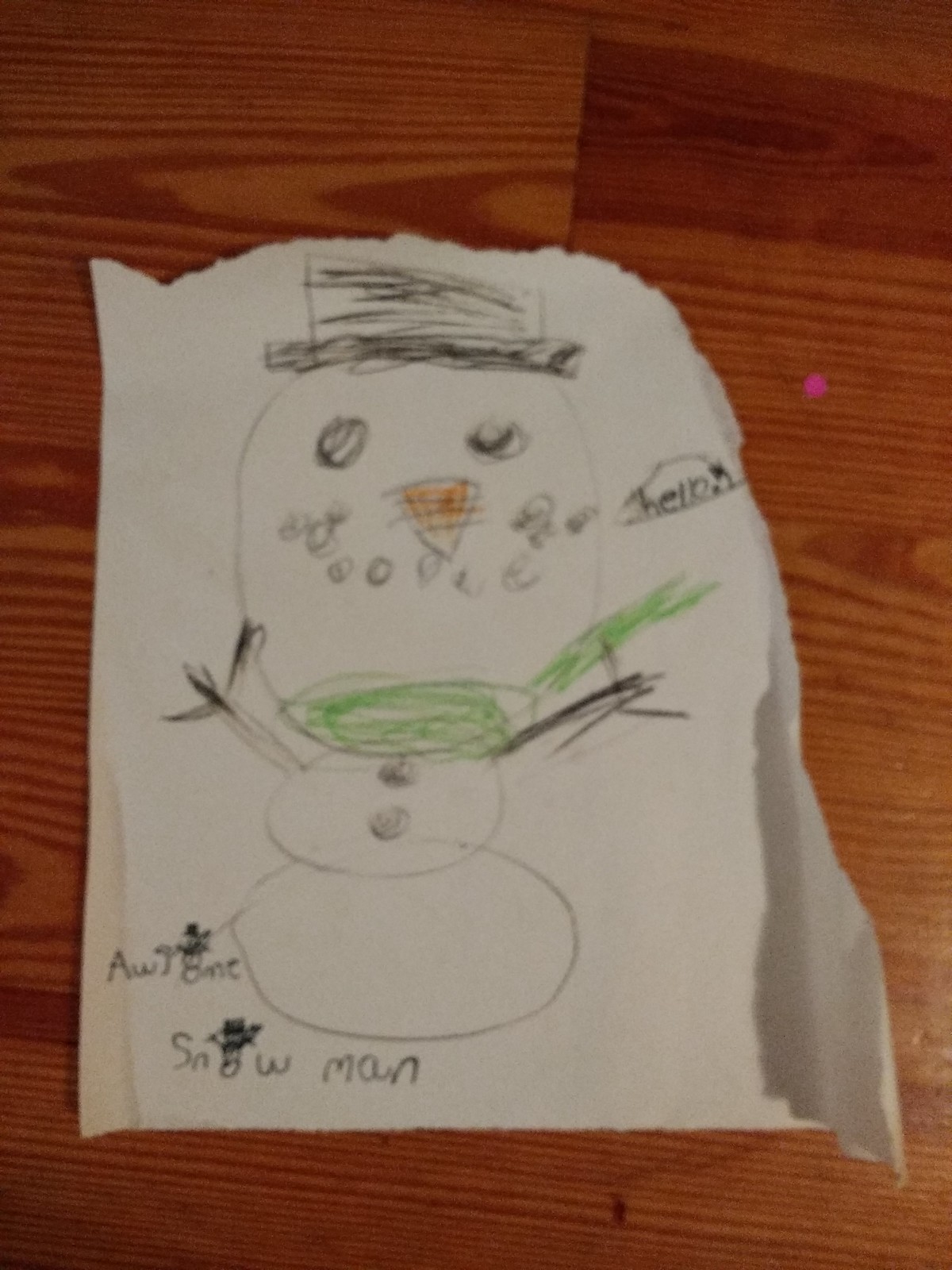This image captures a child's drawing or illustration photographed against a wooden background, possibly a table or floor. The centerpiece is a roughly torn piece of white paper adorned with a charming snowman sketch, predominantly created using colored pencils. The snowman is illustrated with black lines, featuring a green scarf that is somewhat scribbled, a carrot-like orange triangular nose, and eyes and a smile formed by small black dots. Adorning the snowman's head is a classic top hat, also rendered in black. Adding a touch of whimsy, a speech bubble emerges from the snowman's mouth with the word "Help!" written inside, emphasizing the playful nature of the drawing. Towards the bottom of the paper, the word "snowman" is legibly written, accompanied by additional, less discernible writing. The overall impression is one of innocent creativity and the simple joys of childhood art.